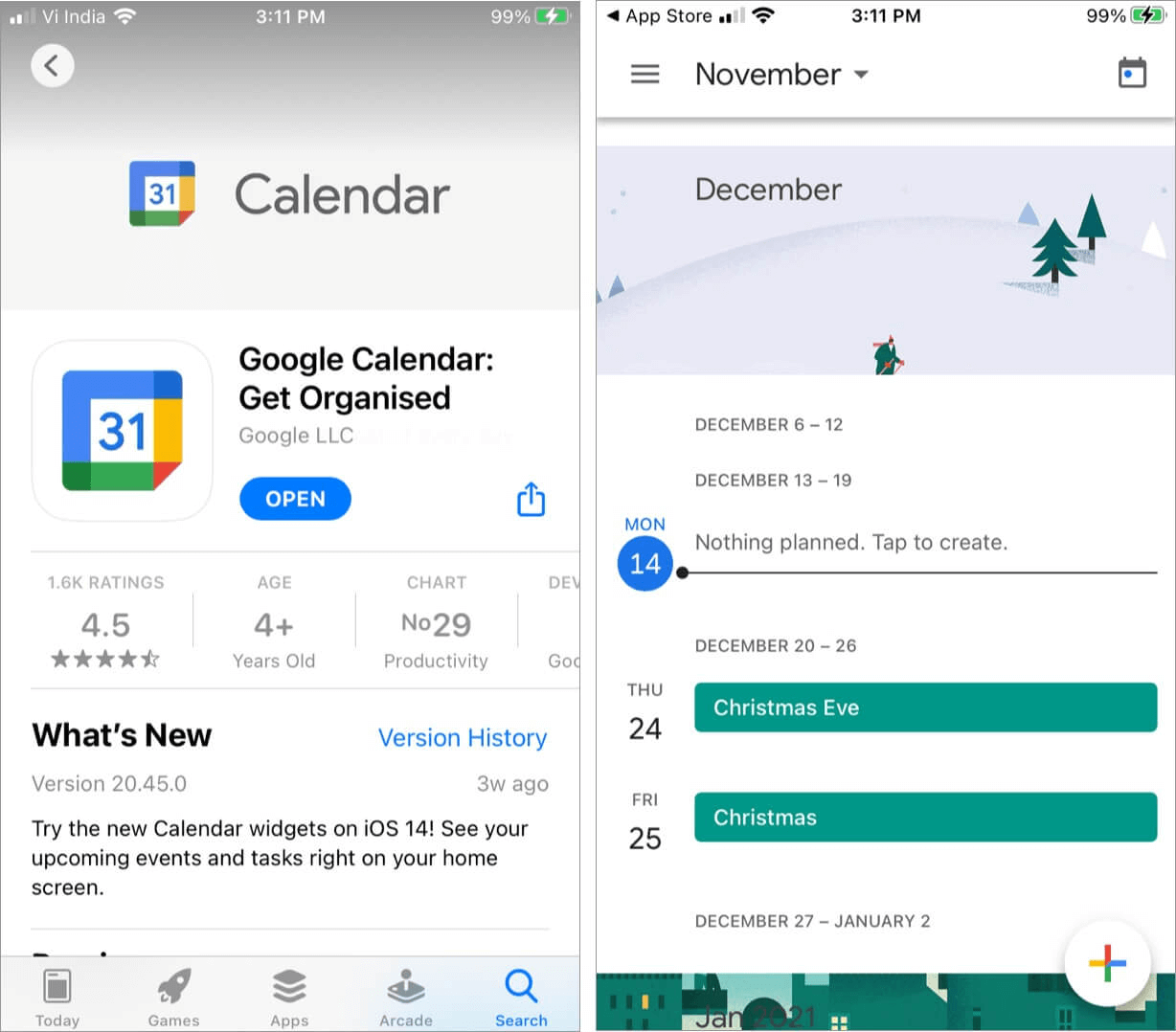**Left Smartphone Screen: Google Calendar App Information:**

The left smartphone screen displays details for the Google Calendar app on the App Store. The background transitions from white at the bottom to light gray at the top. The top bar shows signal strength, "VI India," a Wi-Fi icon, the time (3:11 PM), and battery status at 99% with a green-filled battery icon featuring a white lightning bolt.

Beneath the top bar, there's a gray arrow in a white circle indicating a back function. The app title "Calendar" is centered in large gray letters. Below it is a square icon in Google logo colors: blue (top and left), red (right), and green (bottom), with a corner-turn effect revealing a small red triangle. In the center of the square, a white rectangle with the number "31" in blue signifies the Google Calendar logo.

The screen displays "Google Calendar" and a tagline "Get Organized" using British spelling ("Organise"). Below this, it reads "Google LLC." A blue oblong button labeled "Open" is present with an upload icon (a blue arrow in a blue-outlined square) next to it. 

A thin gray line below shows the app's ratings and details. The app holds 1.6K ratings with an average rating of 4.5 stars, is suitable for users aged 4 years and up, and ranks #29 in the Productivity category. Another thin line separated the section, followed by "What's New" in bold, with "Version History" in blue on the right. The version 20.45.0 updated three weeks ago highlights new iOS 14 calendar widgets for better home screen integration of events and tasks.

At the bottom of the screen, five icons are visible: a calendar labeled "Today," a rocket labeled "Games," a stack labeled "Apps," a joystick labeled "Arcade," and a blue magnifying glass labeled "Search." The "Search" icon and label are blue; the others are green.

**Right Smartphone Screen: Calendar Interface:**

The right smartphone screen also shows a calendar interface with the title "App Store" at the top left, next to signal and Wi-Fi icons. The current time is 3:11 PM and the battery status is 99%.

Below the top bar is a November label with a dropdown to change the month, accompanied by a three-line menu icon on the left and a calendar icon on the right. Underneath, a gray line separates the header from the calendar interface.

A light gray-blue text box displays December, accompanied by an illustration of a skier on a snowy slope with trees in the background. Small text dates range from December 6th to 12th, and December 13th to 19th, with prompt messages "Nothing planned, tap to create." December 14th is highlighted in blue.

Further down, dates from December 20th to 26th are shown, with a long green bar marking Christmas Eve on December 24th and another highlighting Christmas on December 25th. Finally, December 27th to January 2nd is listed at the bottom, partially obscured by a cropped illustration resembling a city scene for January.